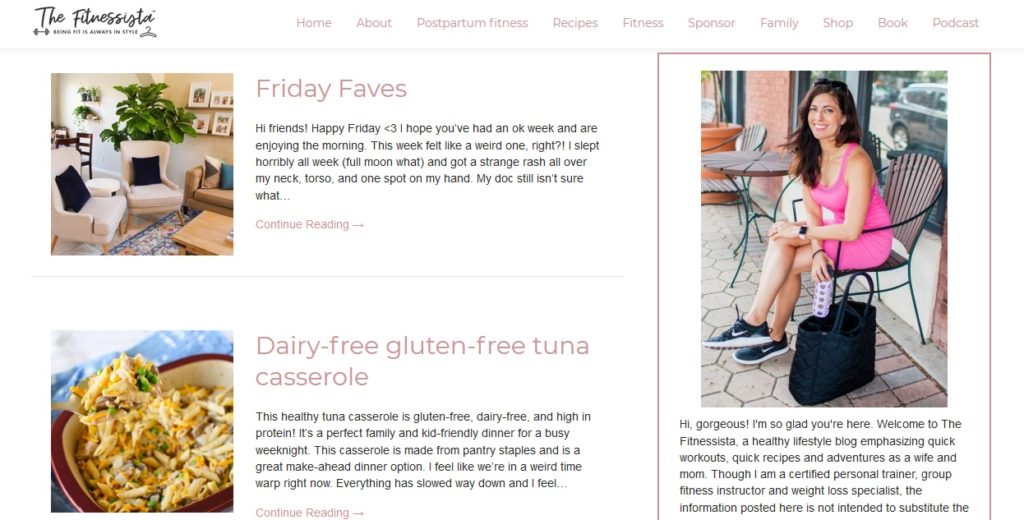This image is a screenshot of the homepage of a website called "Fitnessista," spelled F-I-T-N-E-S-S-I-S-T-A, displayed prominently at the top. The tagline reads "Being fit is always in style," illustrated by a hanger symbolizing style and a pair of weights indicating fitness on the left side. The navigation bar at the top includes tabs labeled Home, About, Postpartum Fitness, Recipes, Fitness, Sponsor, Family, Shop, Book, and Podcast. Below the navigation bar are clickable articles. The first article is titled "Friday Faves" and is accompanied by a picture of a cozy living room. The second article, "Dairy-Free, Gluten-Free Tuna Casserole," is illustrated with an appetizing image of the dish. Additionally, a photograph of the website's creator, seated in a chair holding a bottle of water, is visible, suggesting a personal connection and commitment to the fitness lifestyle presented on the site.